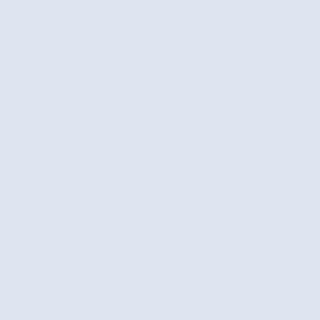The final image in the set depicts a nearly square, rectangular box with a solid, light purple color. It is minimalistic in nature, completely devoid of any content, text, or additional elements. The absence of detail leaves a clean, uninterrupted field of soft purple, exuding simplicity and uniformity. The dimensions suggest a slight rectangular form, but it is very close to a perfect square. Its stark emptiness and monochromatic palette make it a purely abstract representation.